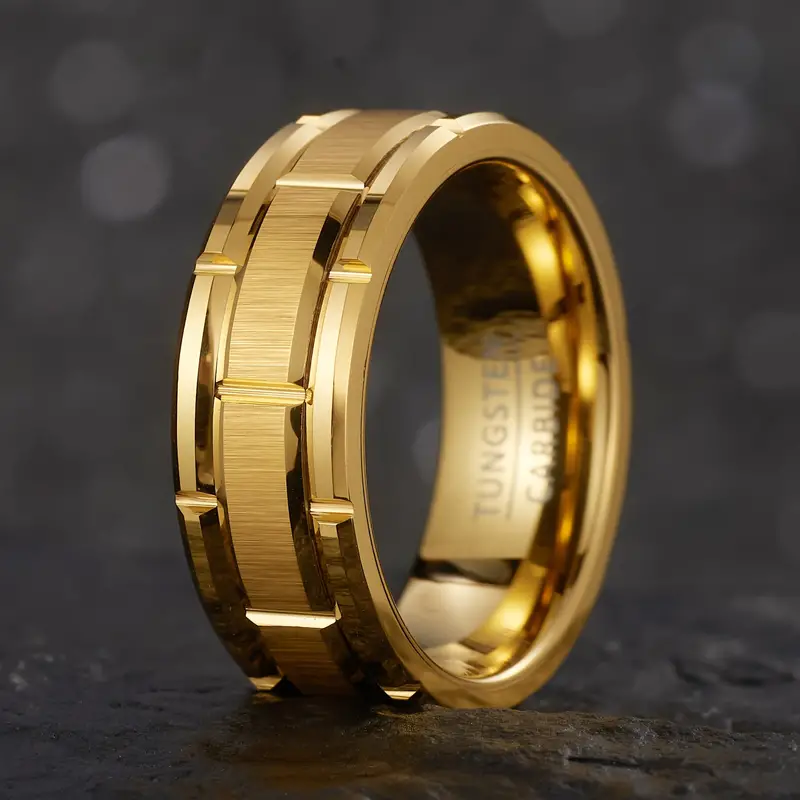The image showcases a heavy, gold-colored tungsten carbide ring prominently positioned upright on a blurred, dark surface, reminiscent of a tire standing on its edge. The ring is intricately designed with three distinct bands: two outer bands and one central band, each featuring symmetrical notches that create a repeating pattern. Inside the smooth, shiny inner band, the words "tungsten carbide" are clearly engraved in white. The lighting accentuates the ring's golden hue and reflective surfaces, making it the focal point against the dark, out-of-focus background.